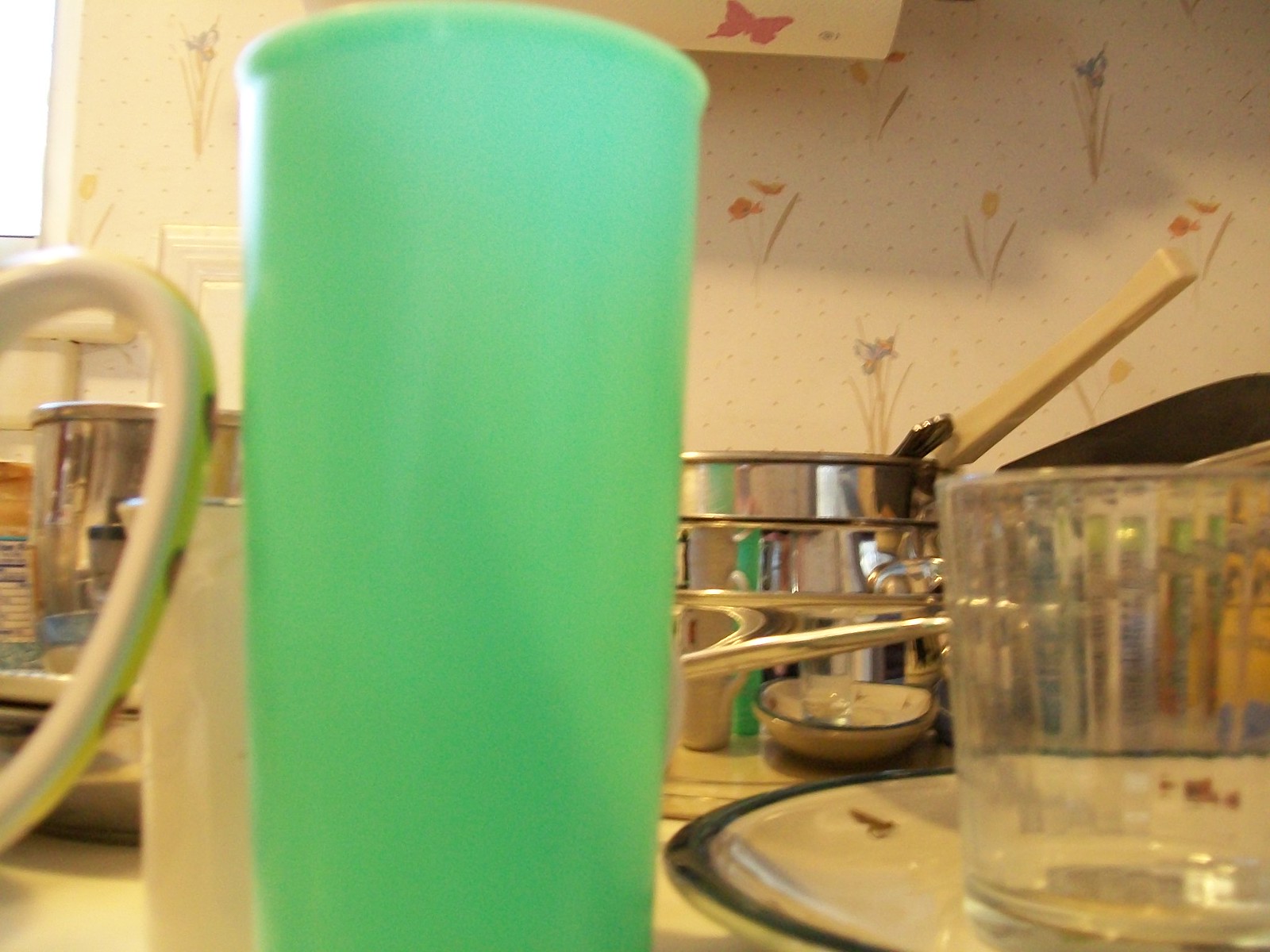The photo captures a bustling kitchen scene from an eye-level perspective, where the camera appears to be placed directly on the countertop. Dominating the foreground is a tall, light green plastic cup, complemented by a short glass cup with distinct grooves to its right, perched atop a white plate. Scattered around are various kitchen essentials including shiny silver pots and pans, a coffee mug with its handle visible on the left, and a mix of scoops and tongs. The minimalistic wallpaper, primarily white and adorned with small dots, flowers, and an occasional butterfly, adds a subtle decorative touch to the backdrop. A window on the left bathes the scene in soft, natural light, casting gentle reflections off the metallic surfaces of the pots and pans.